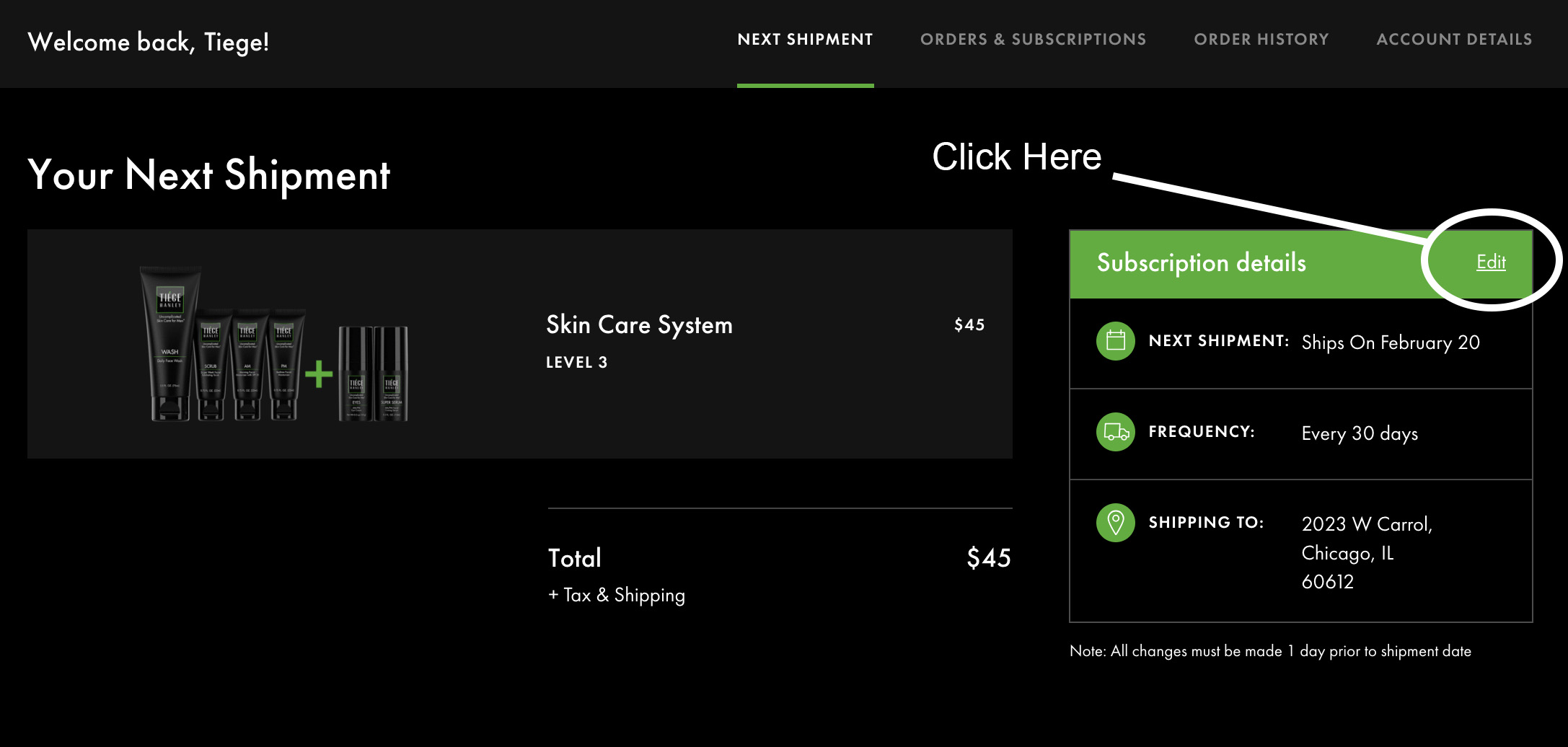The image features a meticulously designed web interface predominantly in dark colors. The main background is black, topped with a gray rectangle. Prominently displayed within the gray bar, a friendly greeting reads "Welcome back, Teagle." Immediately to the right, in white text, it states "Next Shipment," underscored by a green line. In smaller, gray text below, options for "Orders and Subscriptions," "Order History," and "Account Intakes" are listed.

To the right side of the black background, the section is labeled "Your Next Shipment." This section includes a dark gray rectangle containing several visual elements: images of tubes, indicative of a cosmetic or skincare product, a plus sign, and two smaller cylinder-like objects. To the right of this image, the text identifies the product as "Skin Care System Level 3," priced at $45.

Beneath the dark gray area, a gray line spans halfway across, ending with the text "Total $45," which includes a note about tax and shipping. Just above this line, the text "Click here" is highlighted in white, accompanied by a circle that presumably guides users on where to click for more information or to proceed. This area is labeled "Subscription Details."

As part of the user interface, there are three black rectangles, each outlined in light gray. Inside these rectangles, there are three green circles containing line drawings, though the specifics of these drawings are not entirely clear. This section provides important shipping details: the next shipment, scheduled to ship on February 20th, occurs every 30 days and ships to a specified address. Additional information is present beneath these rectangles, though it is too small to be legible in the image.